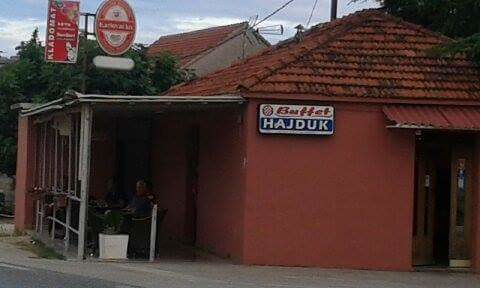This color photograph, taken outdoors on a very cloudy day, depicts a red stucco and brick building with a distinctive red corrugated roof, resembling Spanish tiles. The building fronts a terrace area with railings, where a couple of people are seen sitting at tables, suggesting it might be a local eatery, possibly a restaurant. Above the terrace, there are a couple of red signs, and prominently displayed on the front of the building is the word "buffet," followed by an unclear name. The entrance, a wooden double door with the left side open, adds to the inviting atmosphere. In the background, to the left, green trees and power lines are visible under the overcast sky, along with another tan building with a red roof further off.